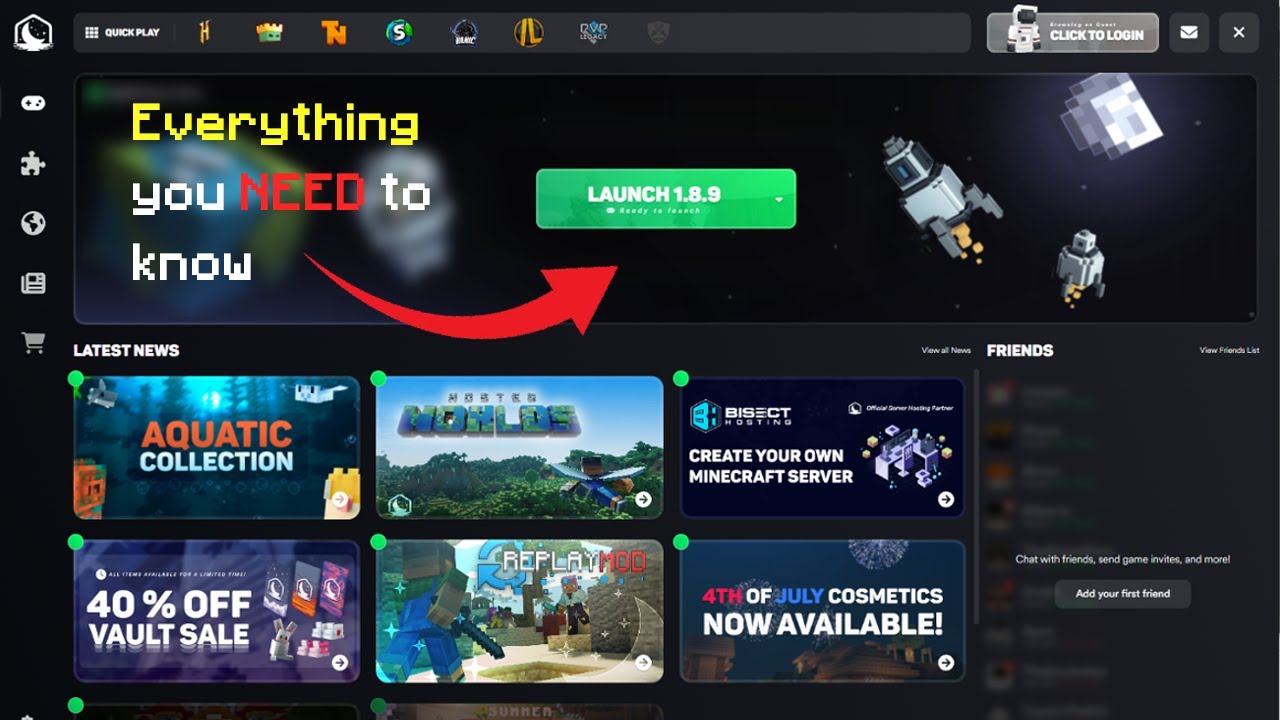The image depicts a dark-themed website interface with a series of icons aligned across the top. Dominating the upper half of the page is a prominent image featuring multiple spacecraft-like structures that appear to be constructed from Lego pieces, positioned on the right-hand side. Adjacent to these spacecrafts is a vibrant green button labeled "Launch 1.89," emphasized by a large red arrow pointing towards it. The text "Everything you need to know" is displayed prominently on the screen, with "Need" highlighted in red, "You too know" in white, and the rest in yellow for emphasis.

Just below this header, there is a section titled "Latest News" that showcases six small tile images. These images include captions such as "Aquatic Collection," "Create Your Own Minecraft Server," a "40% Off Vault Sale," "Indie Game Spotlight," and "4th of July Cosmetics Now Available," each hinting at various content or promotional offers available on the website.

Further down, under a designated "Friends" section, a gray panel provides an option to "Add Your First Friend," accompanied by a conveniently located button just beneath the panel for users to initiate the friend-adding process.